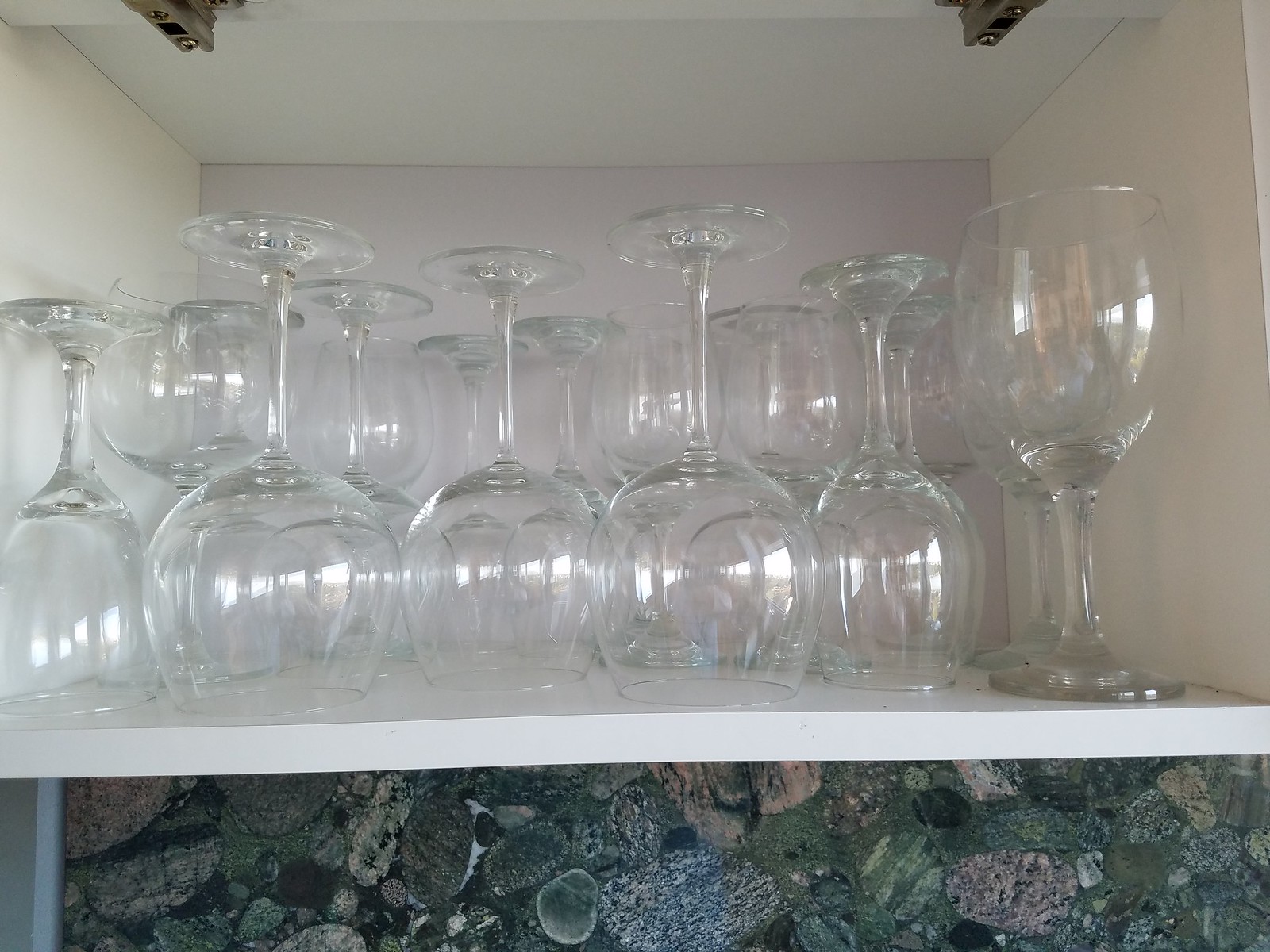This digital photograph, taken indoors, shows an organized display inside a very white cabinet with a wood structure creating a boxed shelf. On this white shelf, there are 18 clear glass wine glasses; the majority are turned upside down with their rims facing downward, while two glasses on the far right are standing upright. The glasses reflect bright sunlight streaming in from nearby windows. Below the shelf, the kitchen backsplash is visible, consisting of a composite rock material with a speckled pattern in shades of grey, green, blue, pink, black, and white. The back wall of the cabinet has a light lavender hue, adding a subtle contrast to the predominantly white setting. Additionally, silver hinges are seen at the top of the cabinet, enhancing the overall modern aesthetic.